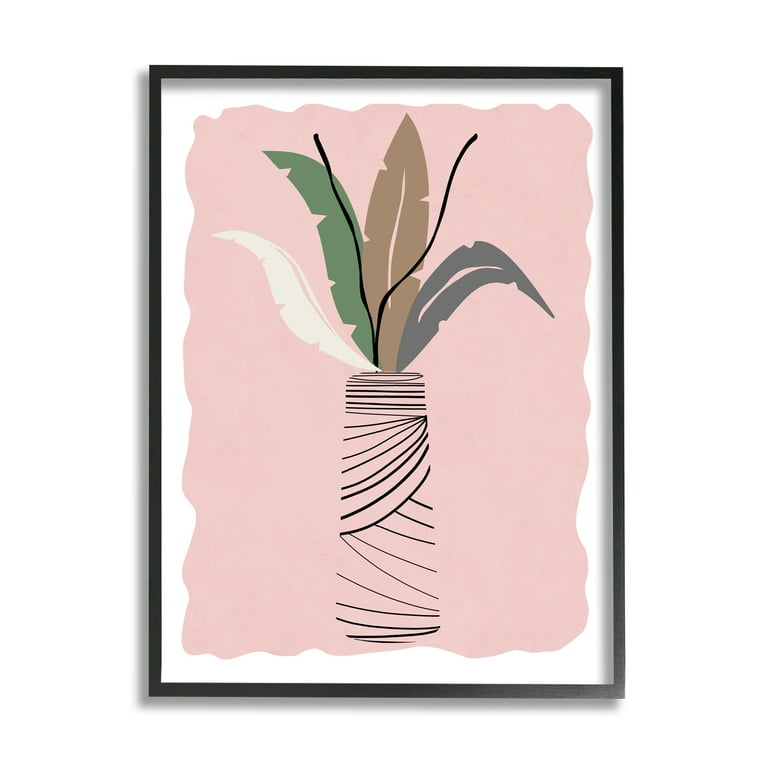This is an image of an abstract painting that features a vase framed by two borders: a solid black outer border and a white inner border. The painting itself rests on a peach or light pink background with jagged edges transitioning into the white border. The vase is created with black horizontal lines and diagonal lines emanating from the middle, enhanced by a horizontal zigzag at the base. Inside the vase, which gives a poster print appearance, there are various leaves. From left to right, a white leaf extends from the middle towards the upper left, a green leaf reaches from the center to the upper left corner, a brown leaf points vertically upwards, and a gray leaf curves up and then down towards the right middle. Additionally, two black V-shaped tendrils rise from the middle of the vase. In the bottom and left parts of the image, a shadow of gray complements the digital representation of the painting. The overall color scheme predominantly features pink, black, white, gray, and green accents.